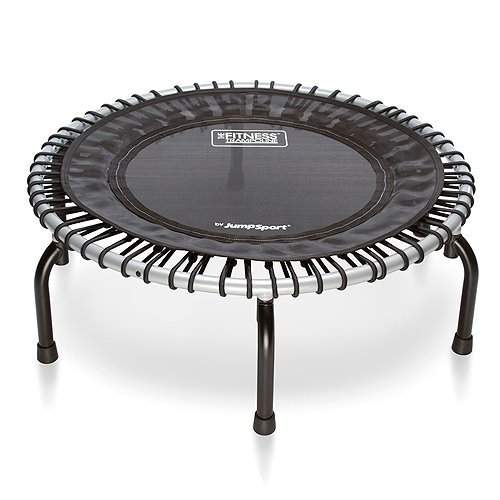This image displays a small, round, individual-sized trampoline set against a clean white background. The trampoline features a silver or white circular metal frame supported by six black legs, three of which are visible in the foreground. Attached to the frame are numerous black straps that connect it to the central black fabric mat. This mat has a slightly shiny finish and a darker black border. At the top of the mat, a white rectangular box contains the text "Fitness Trampoline," and at the bottom, the logo "Jump Sport" is prominently displayed in white. The overall condition of the trampoline appears to be clean and well-maintained.